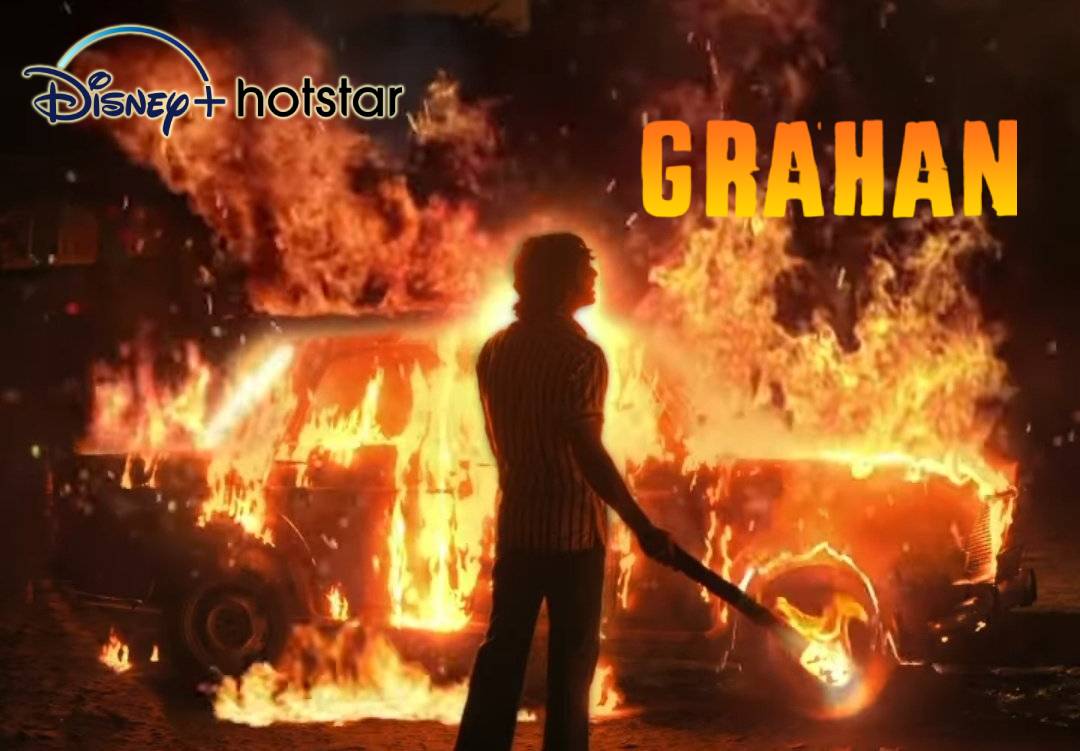The image depicts a striking and intense scene that seems to be a promotional poster for a show, likely on Disney Plus Hotstar. In the top left corner, there are logos for Disney Plus in dark blue and Hotstar in black with a white outline. The top right corner features the name "GRAHAN" in a gradient of light to dark orange letters, evoking the look of flames. Central to the image, a person stands in front of a vehicle that is entirely engulfed in fire, with flames so intense that the ground is also ablaze. The person, wearing a striped shirt and blue jeans, holds a torch or flamethrower, with the torch still alight, indicating they may have just set the car on fire. The individual is staring to the right of the vehicle, though their facial expression remains indiscernible. The scene is set against a dark, nighttime backdrop, which highlights the dramatic and perilous nature of the image.